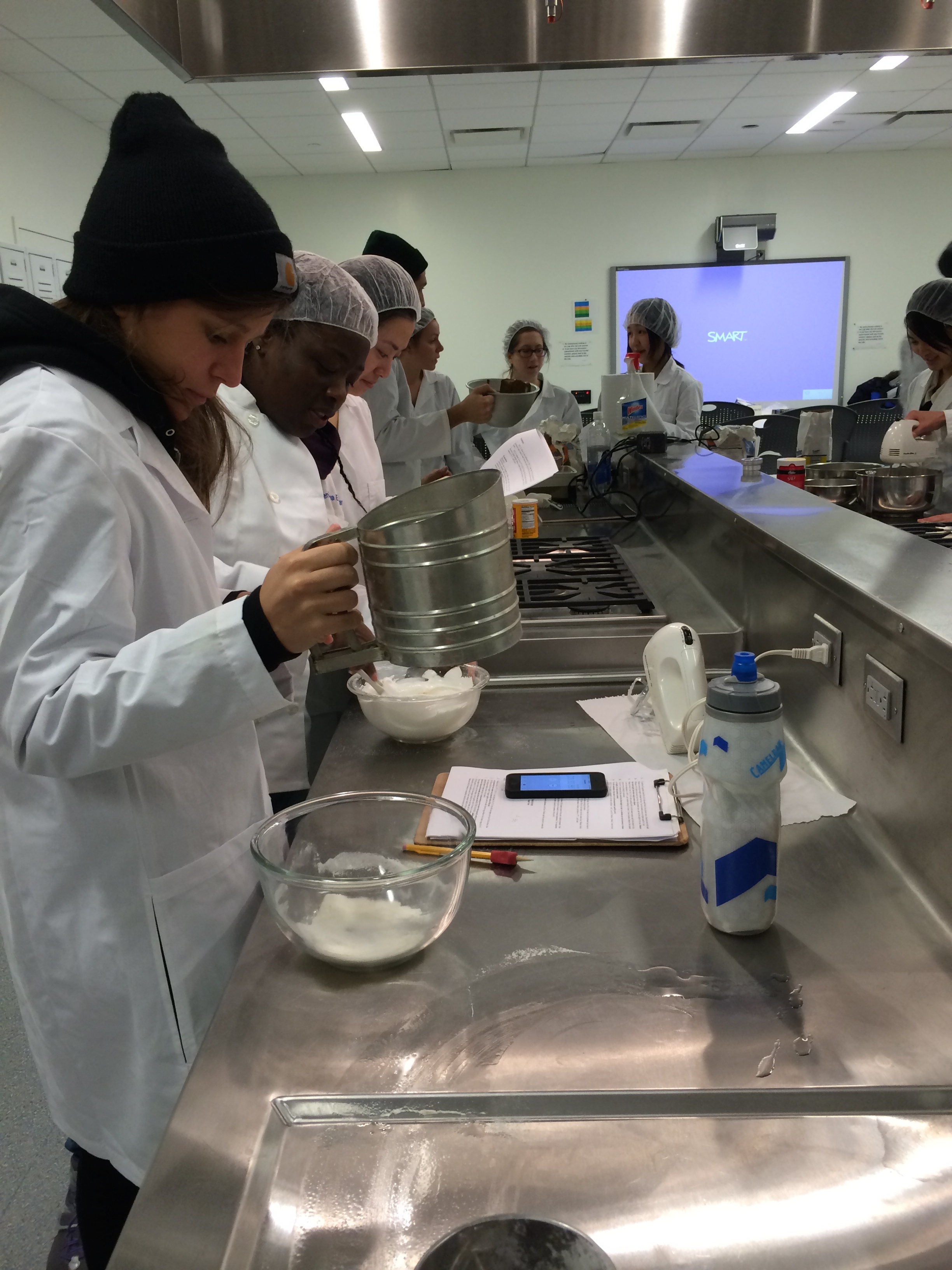The image depicts a bustling chef's kitchen in what appears to be a culinary institute or a cooking class. Several individuals, predominantly women, are lined up along a stainless steel countertop that houses a gas stove, with burners situated centrally. The participants are all dressed in white chef's robes or lab coats and have their hair covered with either hairnets or caps; notably, the woman at the forefront sports a winter cap. She is engaged in sifting flour into a glass bowl containing a white powder, possibly flour or sugar. The countertop is adorned with various items including a clipboard with a notebook, a smartphone, a pencil, and a blue and white plastic water bottle. Electrical outlets are visible on the wall behind the counter, and there is a blank computer screen with indecipherable text in the background. The scene portrays a hands-on culinary exercise, with a few more participants in the background, all focused on their cooking tasks.